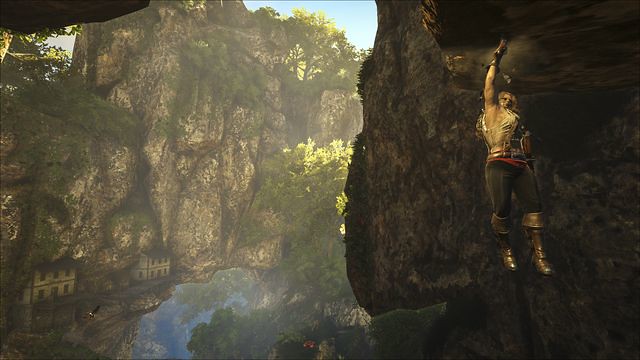In this highly realistic video game screenshot, the scene captures the intense moment of a muscular character clinging to the edge of a towering mountain ledge with just one hand. The character, dressed in rugged gear including brown boots and black pants, displays remarkable strength and determination. On the right-hand side of the image, the precarious ledge juts out dramatically against the backdrop of the expansive mountain landscape. To the left, a towering mountain covered in dense trees rises majestically, leading the eye down to a quaint village nestled at its base. The village, with its scattered buildings, appears to be a serene sky village, providing a stark contrast to the tension and peril experienced by the character on the ledge.